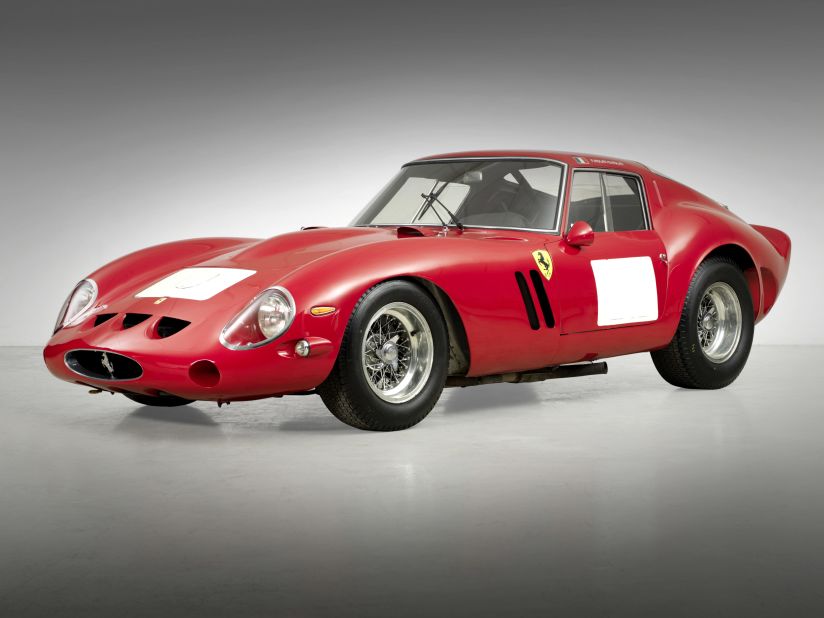A striking photograph captures a vintage, candy apple red sports car, primarily viewed from the side with the front facing slightly left. This classic two-door vehicle, reminiscent of the 1960s, boasts large, oversized black tires with chrome rims. The car's sporty design includes distinct features such as a white rectangular decal on the driver's side door and a matching white rectangle on the hood. A closer inspection reveals an engaged windshield wiper on the driver’s side and dark interior seating material, though precise details are hard to discern. Notably, the car's front showcases three prominent vent-like indents below the hood and a horizontally placed, black-colored oval emblem on the bottom of the bumper. Adding to its nostalgic charm, a yellow shield with a black silhouette of a horse is visible just left of the door, hinting at a possibly Porsche-inspired design.